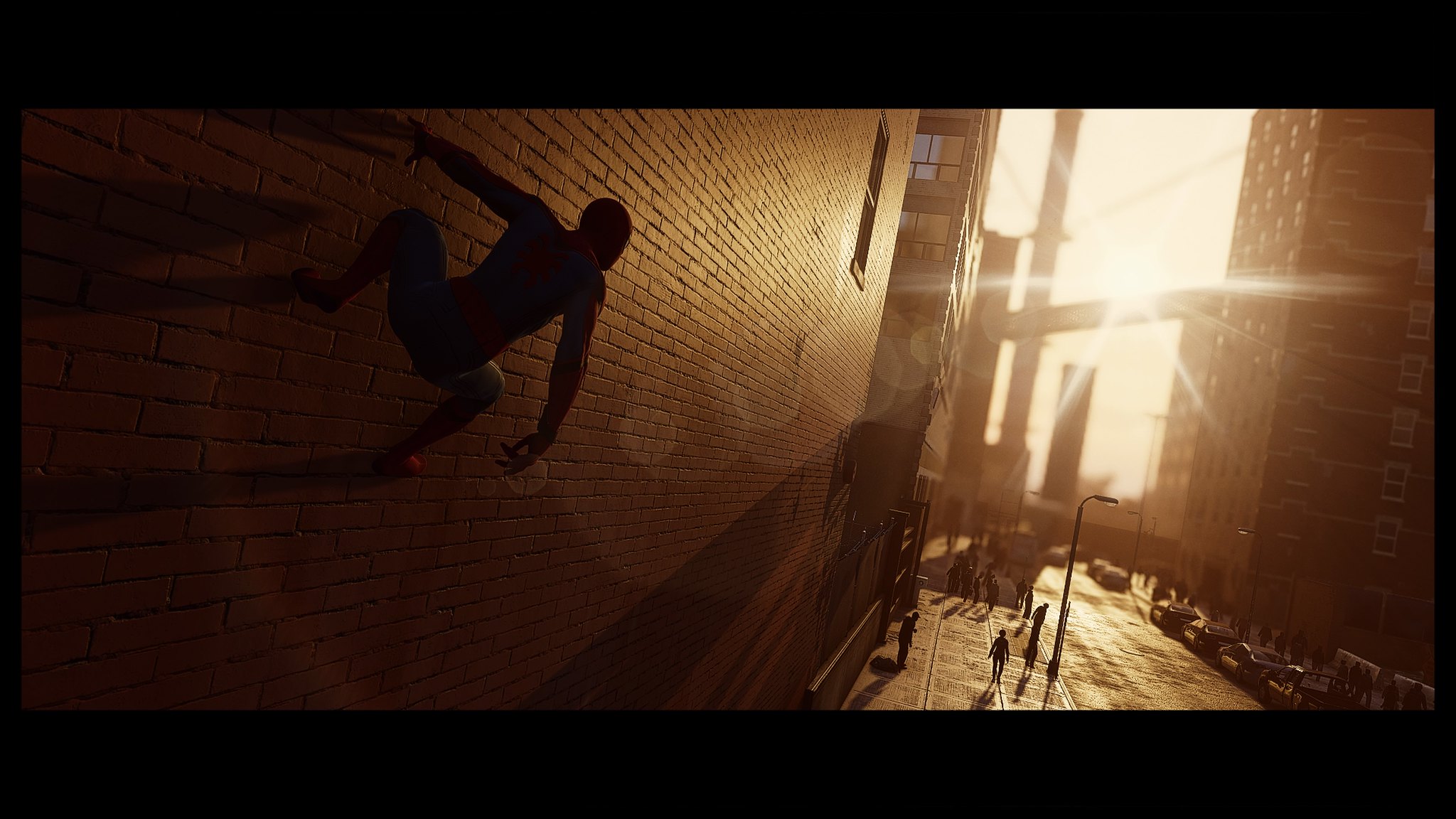In this vibrant scene, seemingly extracted from a video game or animated cartoon, the focal point is a towering brick building on the left side of the frame. Clad in an iconic Spider-Man costume, a character presumed to be Spider-Man is shown clinging to the building's facade with his left arm and both legs firmly planted, while his right arm dangles freely. A window punctuates the front of the brick structure, adding architectural detail.

Beyond this building, a gap reveals another tall edifice adorned with multiple windows, contributing to the urban landscape. The middle of the image showcases a bustling skyline with a bright sun dominating the horizon, casting a luminous glow over the scene. To the right of the sun, an array of additional brick buildings with numerous windows extend the cityscape further.

At street level, a pavement hosts a scattering of indistinct pedestrians navigating the sidewalks. Curved street lamps line the pathway, subtly illuminating the scene despite their small size. While the people's features remain undefined, their presence animates the urban environment, adding a sense of lively activity to the backdrop.